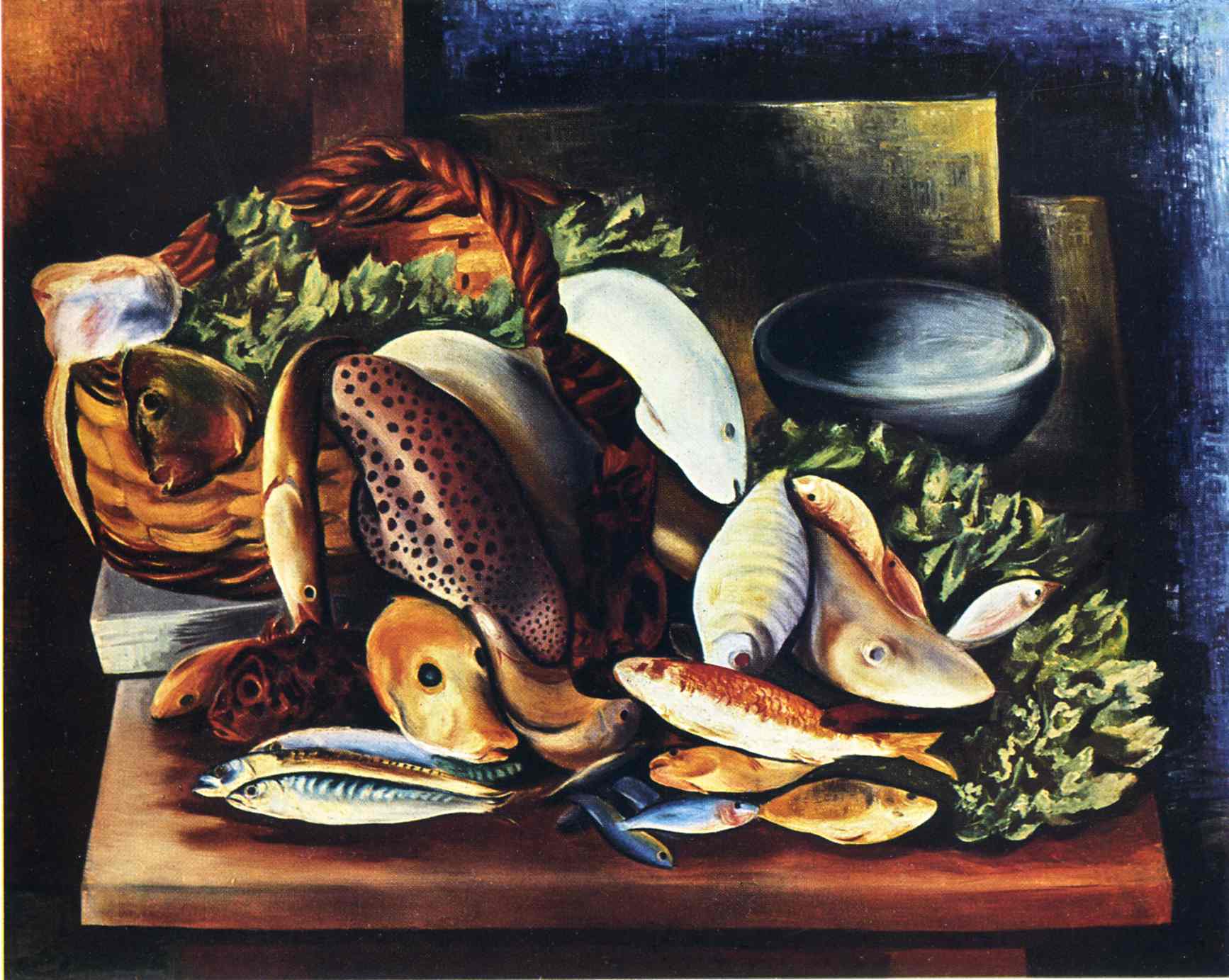The painting depicts a collection of diverse fish piled atop a small wooden table. The arrangement showcases fish of various sizes and colors, with some notable descriptions: a trout with a blue top and yellow bottom, a fish with an orange face and black eyes resembling a dog, and a white fish with black stripes and a yellow streak with red eyes. On the right side, there's a fish with an orange and white body facing right and one turned on its side. Underneath and around the fish, there is green vegetation that resembles lettuce. Nestled among the greenery is a partly visible blue bowl with a white and dark blue interior. Behind the fish sits a wicker basket filled with foliage, featuring a handle arching above it. The background features a gradient blue wall, darker in the center and gradually lightening towards the edges, with some indistinct shapes and colors adding to the composition. The overall scene suggests a preparatory arrangement, enhanced by the semi-realistic art style.